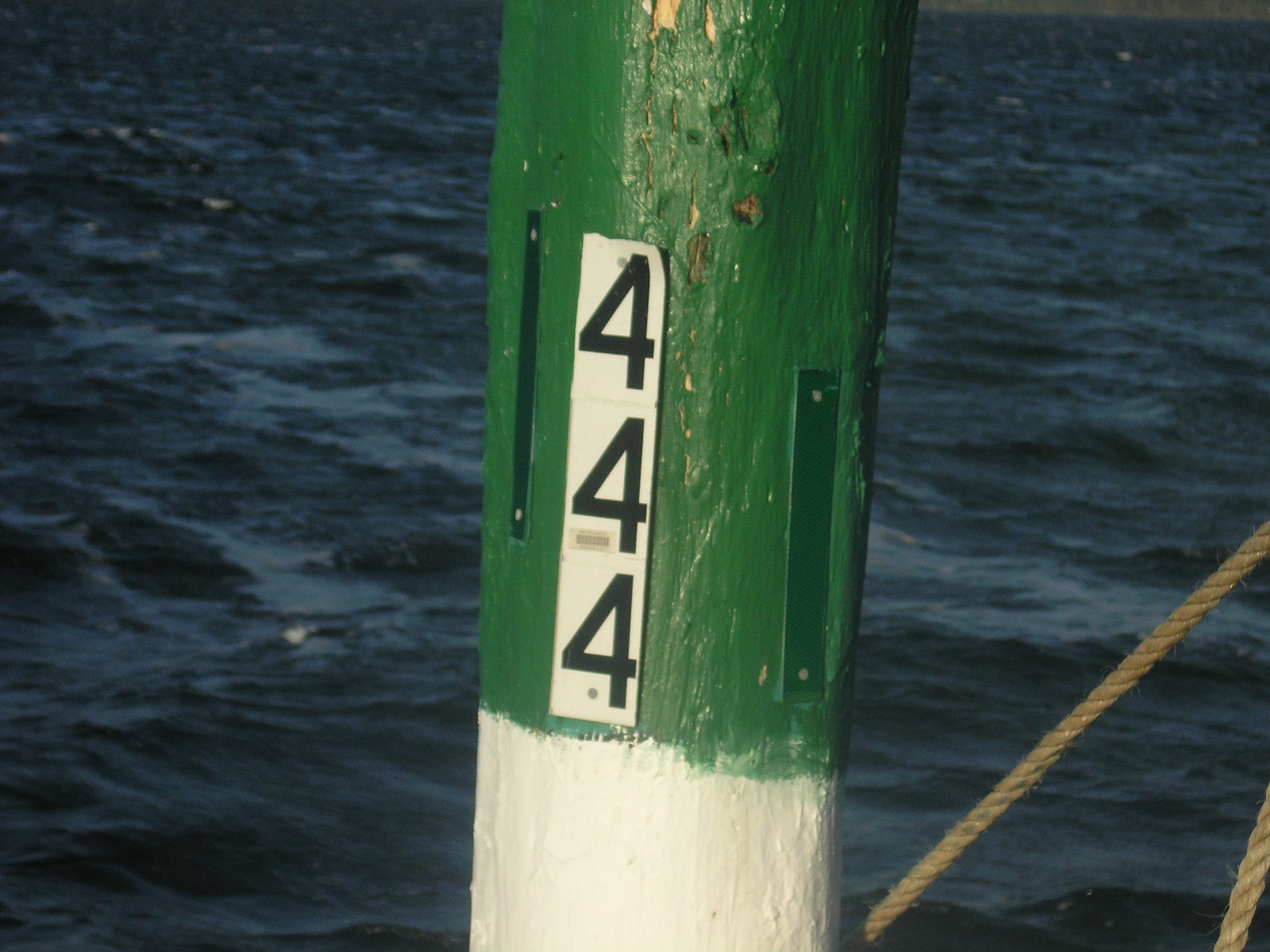The color photo, taken outdoors during the day, captures a close-up of a wooden mooring dock pole near a vast expanse of ocean water. The middle-focused image shows the bottom half of the pole painted white, while the top half features a fading green paint. Emblazoned vertically down the side of the pole are the numbers "444." In addition to these details, there are two dark green metal brackets affixed to the pole. Towards the right side of the photo, a rope extends from the bottom and off to the side, adding to the nautical context of the scene. The background is dominated by the serene blue of the ocean, leaving the exact location—whether a boat, dock, or deck—ambiguous.